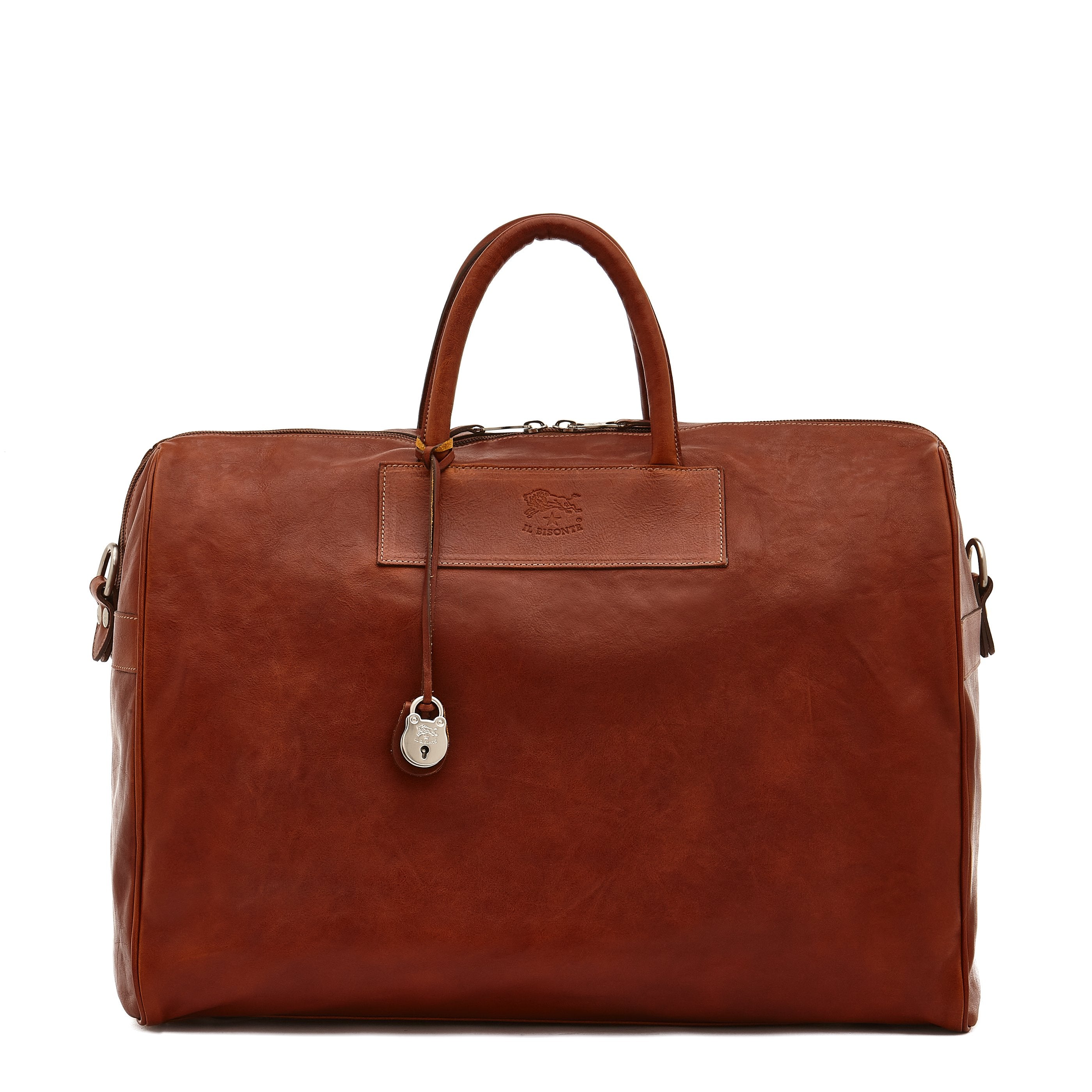This photograph showcases a highly detailed men's leather travel bag by Bisante, featuring a rich reddish-brown color and soft-sided construction. The bag has a distinct unisex appeal, with the Bisante logo prominently displayed below the handle, featuring a leaping bull above a star, intricately engraved into the leather. The bag is equipped with dual soft handles on either side of a double zipper, ensuring ease of carrying and accessibility. A striking feature is the beautiful leather strap with a silver padlock hanging down the side, adding both a stylish touch and practical functionality. The bag's design allows it to also function as a versatile handbag, suitable for carrying a laptop and other essentials.